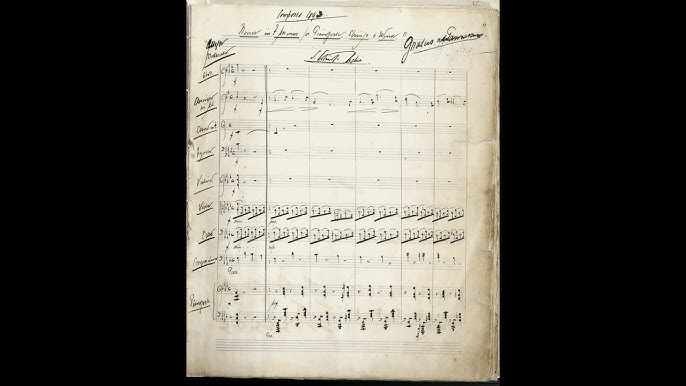The image depicts a piece of aged and weathered sheet music, with a prominent yellowish tinge indicating its vintage nature. The edges of the paper are tattered and discolored, with noticeable wrinkling especially on the right, top, and left sides. The background surrounding the sheet music is solid black, suggesting the image might have been scanned and cropped this way. The content itself consists of handwritten musical notes and hurried cursive text, though the precise words are too small to discern. The paper's layout features multiple lines of music, some of which contain notes while others are blank or minimally filled. The noticeable sections of cursive are scattered, particularly at the top and the left margin. Overall, the piece presents a nostalgic yet enigmatic artifact, capturing the tactile history of a hand-drawn composition.